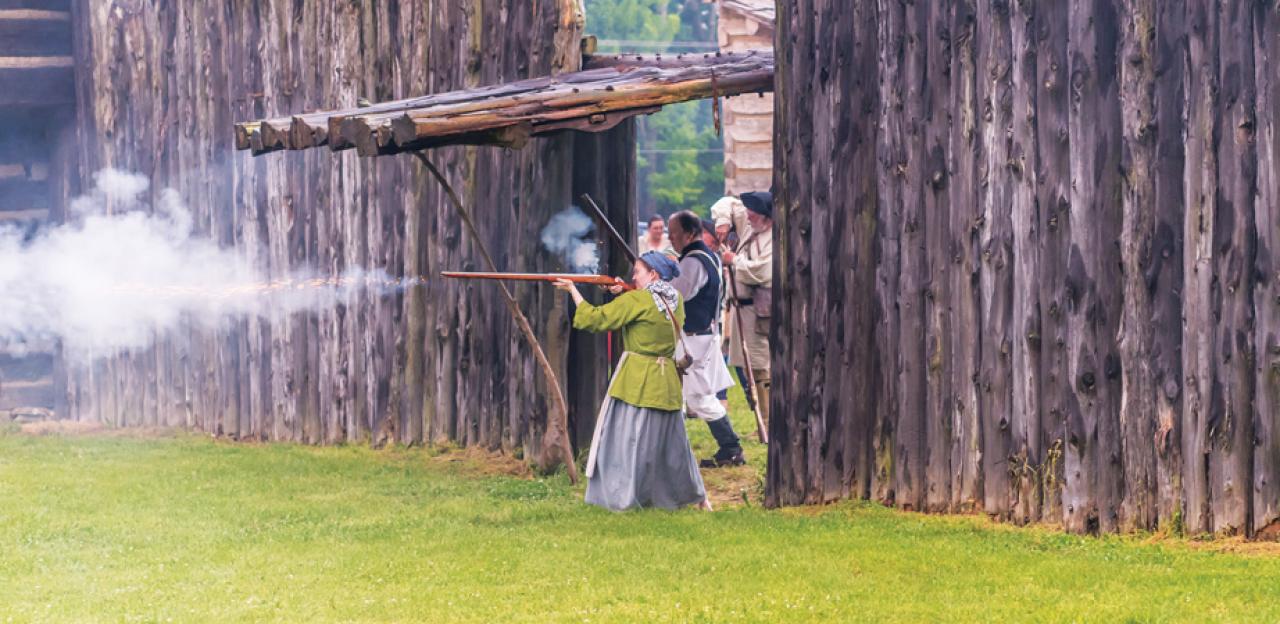This image captures an angled view of a historical battle reenactment taking place beside a large wooden fort. The fort's log walls are both to the left and right, extending out of the frame, and feature a sizable, propped-up log door held by branches, through which you can see several performers in period costumes. Foregrounded against the green grass, a woman in a long grey skirt, green long-sleeved top, and blue head kerchief stands under the lifted door. She is firing an old-fashioned shotgun, with visible smoke billowing from the barrel. Behind her stands a man dressed in medieval garb consisting of white pants, black boots, a white shirt with suspenders, and a blue vest. He also appears to be shooting a rifle, evidenced by the smoke trailing from his gun. In the distant background, more reenactors can be glimpsed through the open fort door, adding to the rich historical tableau.